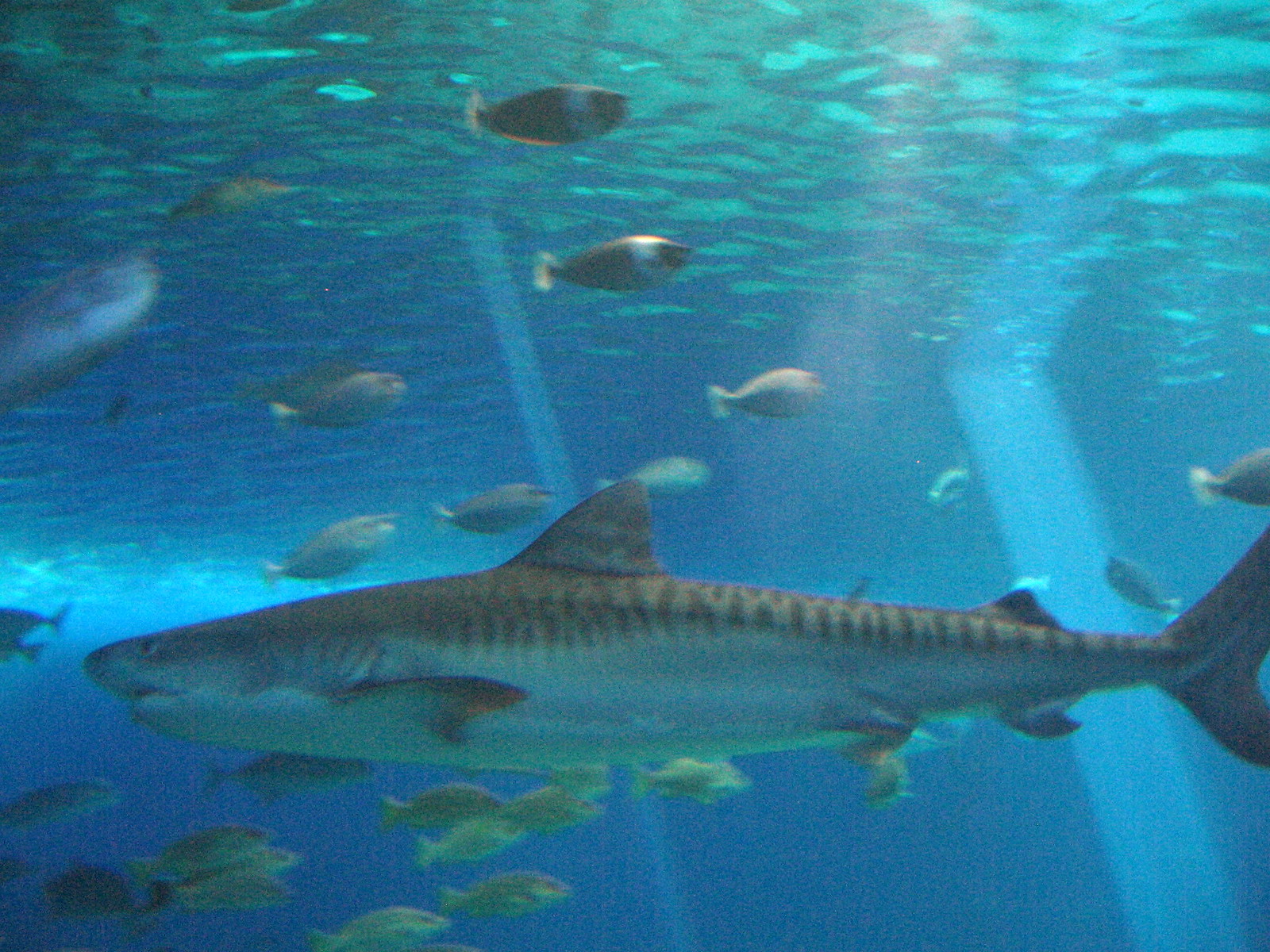This detailed image depicts a large public aquarium, with an underwater scene bathed in blue light and hints of green. The composition captures the dynamic contrast between marine life moving in opposite directions. Dominating the center of the scene, a large shark, identifiable by its gray body, lighter underbelly, and distinctive stripes across its back, top fin, and tail fin, swims leftward. Surrounding it, numerous small, round, and oval-shaped fish, mainly light gray, drift rightward. A medium-sized fish, also gray, can be seen above the shark, swimming upward. Sunlight filters in from the top, illuminating the water and casting mesmerizing shadows, suggesting the photo was taken from within an indoor aquarium. The observer’s perspective appears level with the marine creatures, enhancing the immersive experience.